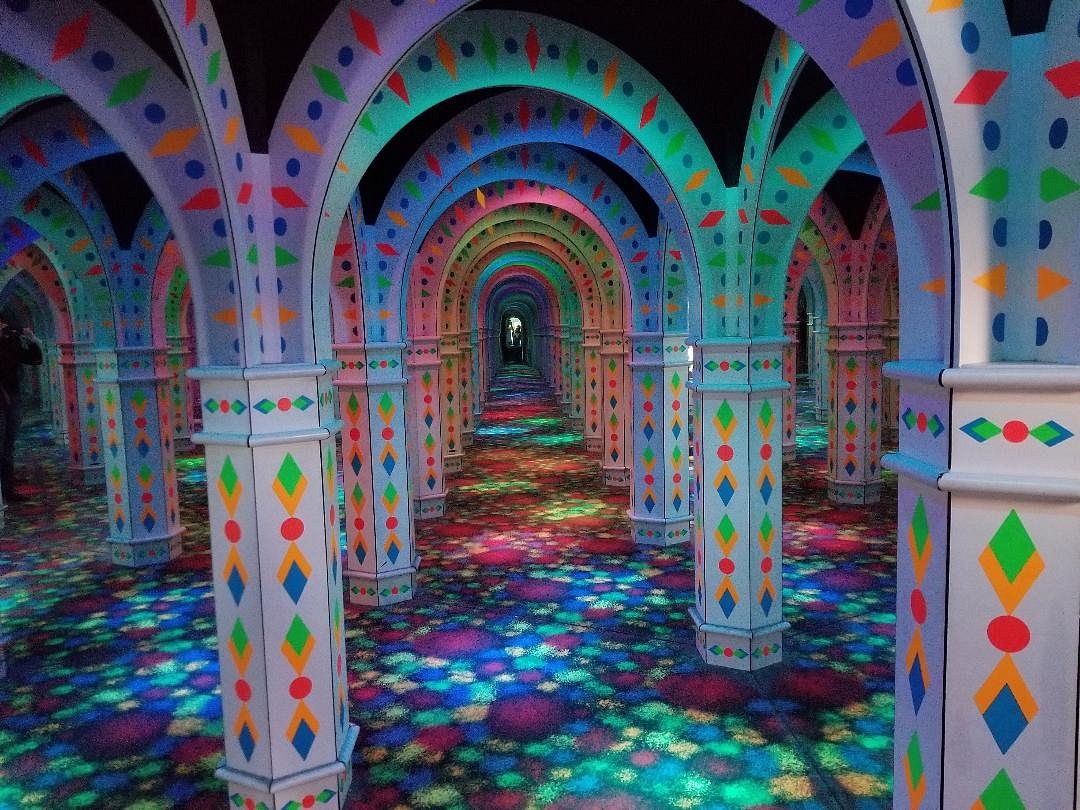The image portrays a mesmerizing, seemingly endless corridor composed of numerous arches and hexagonal columns adorned with intricate diamond and circular patterns. Each archway is painted white and repeatedly decorated with a prominent green on top, yellow on the bottom diamond with a red dot, followed by another diamond painted yellow on top and blue on the bottom. This decorative motif extends along the length of the hallway. The multicolored floor complements the vivid columns, covered in a mosaic of green, yellow, red, and blue dots, creating a psychedelic and strobe-like effect. Far off in the distance, the hallway seemingly concludes with a faint light and what appears to be a statue or bust, though it's discernibly unclear due to the immense depth. The architectural design evokes the sense of a colossal, intricately decorated basement or a fantasy setting for a game like laser tag, characterized by a surreal and otherworldly ambiance.